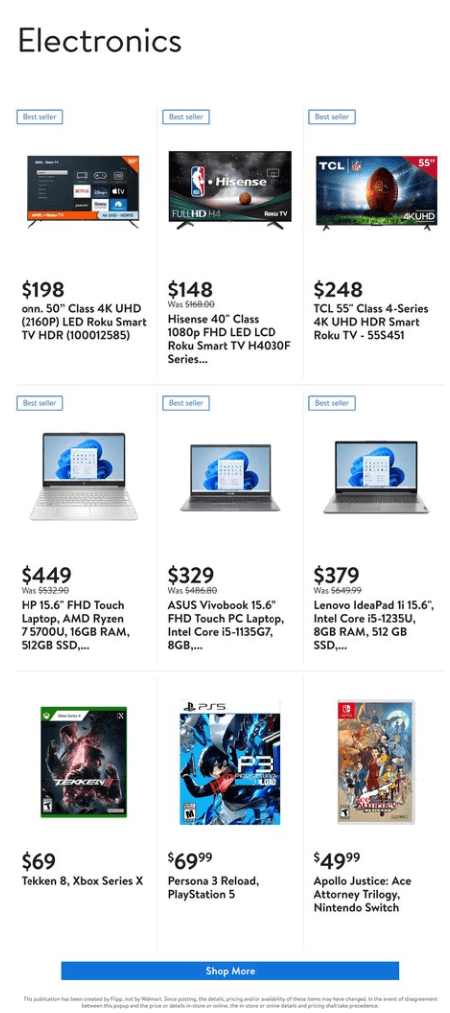In the top left corner, various electronics are showcased with the word "Electronics" displayed in black digital font. Featured prominently is a 50-inch class 4K UHD LED Roku Smart TV (model: 100012585), labeled as "ON." Moving to the right, there is a Hisense 40-inch class 1080p FHD LED LCD Roku Smart TV (model: H4030F series) priced at $148. The screen displays an MLB logo with "Hisense" in white lettering and a "Bestseller" tag on top.

Next, at $248, is a TCL 55-inch class 4-Series 4K UHD HDR Smart Roku TV (model: 555451). The screen shows a ball in the bottom right corner, "UHD" at the top left, and "TCL" branding. This model also bears the "Bestseller" distinction.

Below, a row of laptops is displayed, starting with an HP 15.6-inch FHD Touch Laptop, featuring an AMD Ryzen 7 processor (model: 5700U), 16GB RAM, and a 512GB SSD, priced at $449. Adjacent to this, another laptop, slightly darker in color, is marked at $329 as an Asus VivoBook 15.6-inch FHD Touch PC Laptop, equipped with an Intel Core i5 processor (model: 1135G7) and 8GB RAM.